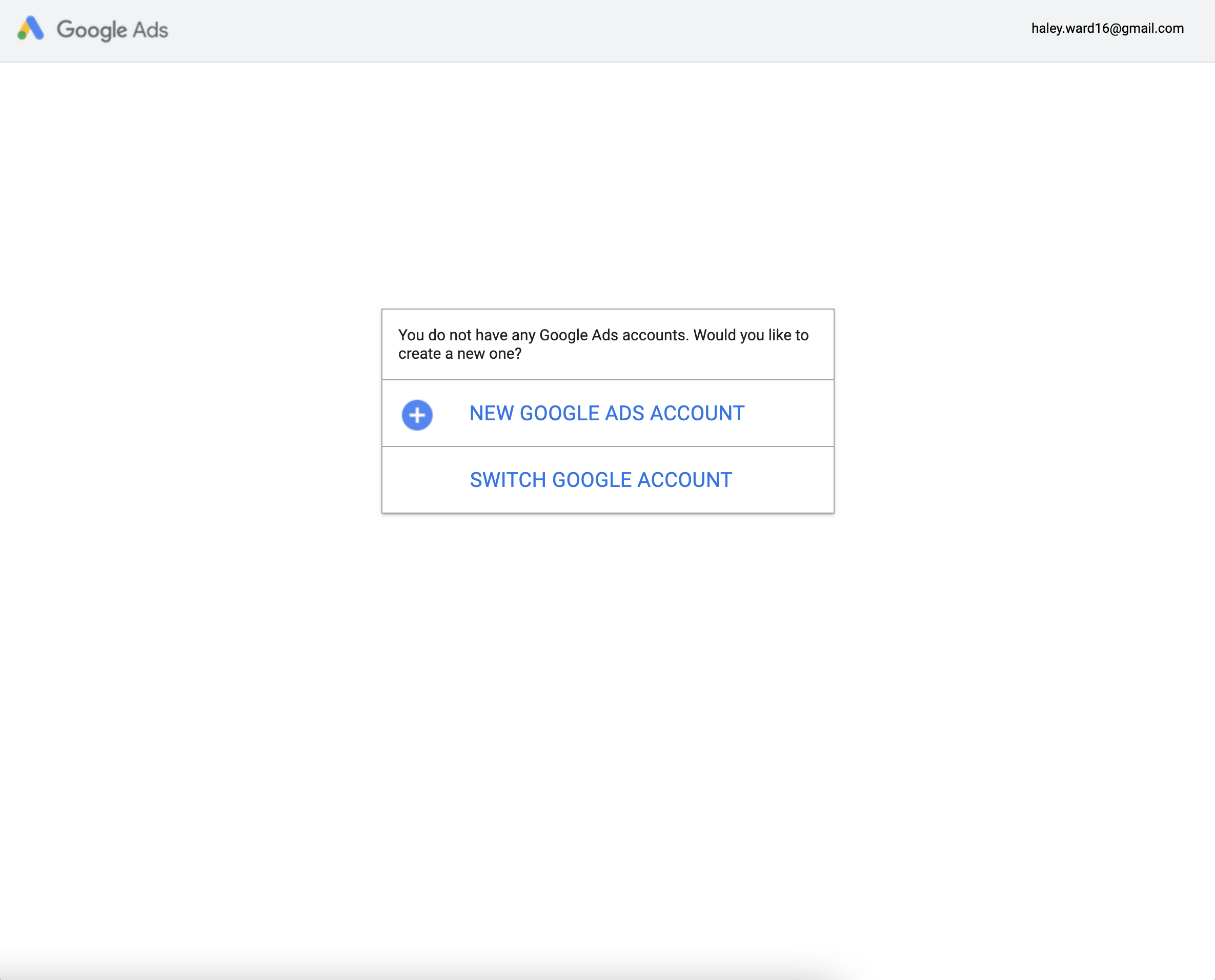This image is a screenshot of a Google Ads website with a predominantly white background. The top border of the website is a very light gray. On the left side, written in a gray font, is the text "Google Ads," adjacent to the Google Ads logo, which is a triangle composed of the Google colors: red, yellow, orange, green, and blue. On the top right side of the screenshot, the email address "hayley.ward16@gmail.com" is displayed.

In the center of the image, there is a lightly outlined rectangle in very light gray. The headline within the rectangle reads, "You do not have any Google Ads accounts. Would you like to create one?" Below this message, there are two options. The first option is written in blue, all capital letters: "NEW GOOGLE ADS ACCOUNT." To the left of this option, there is a blue circle featuring a white plus sign. The second option, located just beneath the first, also in blue text, reads, "Switch Google account."